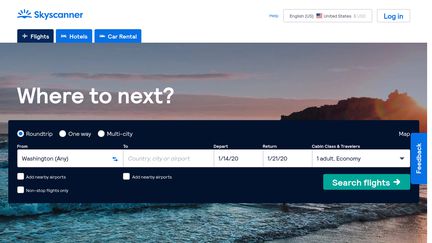**Detailed Caption:**

The image is a landscape-oriented screenshot of the Skyscanner website, displayed as it would appear on a monitor or laptop screen, rather than on a mobile device. In the top left corner of the screen, the Skyscanner logo is prominently featured. The logo consists of blue sun rays rising above blue mountains, accompanied by the site name "Skyscanner" written in bold, sans-serif font with only the initial "S" capitalized.

On the top right corner, there is a "Login" button with "Login" written in blue and outlined by a light gray rectangle. Next to the Login button, there is a longer rectangular region which appears to contain a small US flag icon, but the text inside is too small to decipher; it might be a search box or language selection tool.

Below the top navigation bar, a white blank space dominates most of the screen’s width. On the left side within this blank space, there are three tabs: "Flights," "Hotels," and "Car Rentals." The currently selected tab is "Flights," which is distinguished by a dark blue color, whereas the other two tabs, "Hotels" and "Car Rentals," are in lighter blue shades, indicating that they are not selected.

With the "Flights" tab selected, a screen-wide photo is displayed beneath the tabs. The photo captures a scenic sunset sky above ocean waves gently crashing onto a beach. Spanning the entire width of this image is a large, dark blue search box that matches the color of the selected "Flights" tab. The title "Where to next?" is displayed in large white letters above the search box. The search box itself allows users to input their departure and arrival destinations, among other flight search details.

Below the input fields, there is a white "Search flights" button. Additionally, on the right side of the screen, there is a vertical blue button labeled "Feedback," providing users an option to offer their feedback on the website.